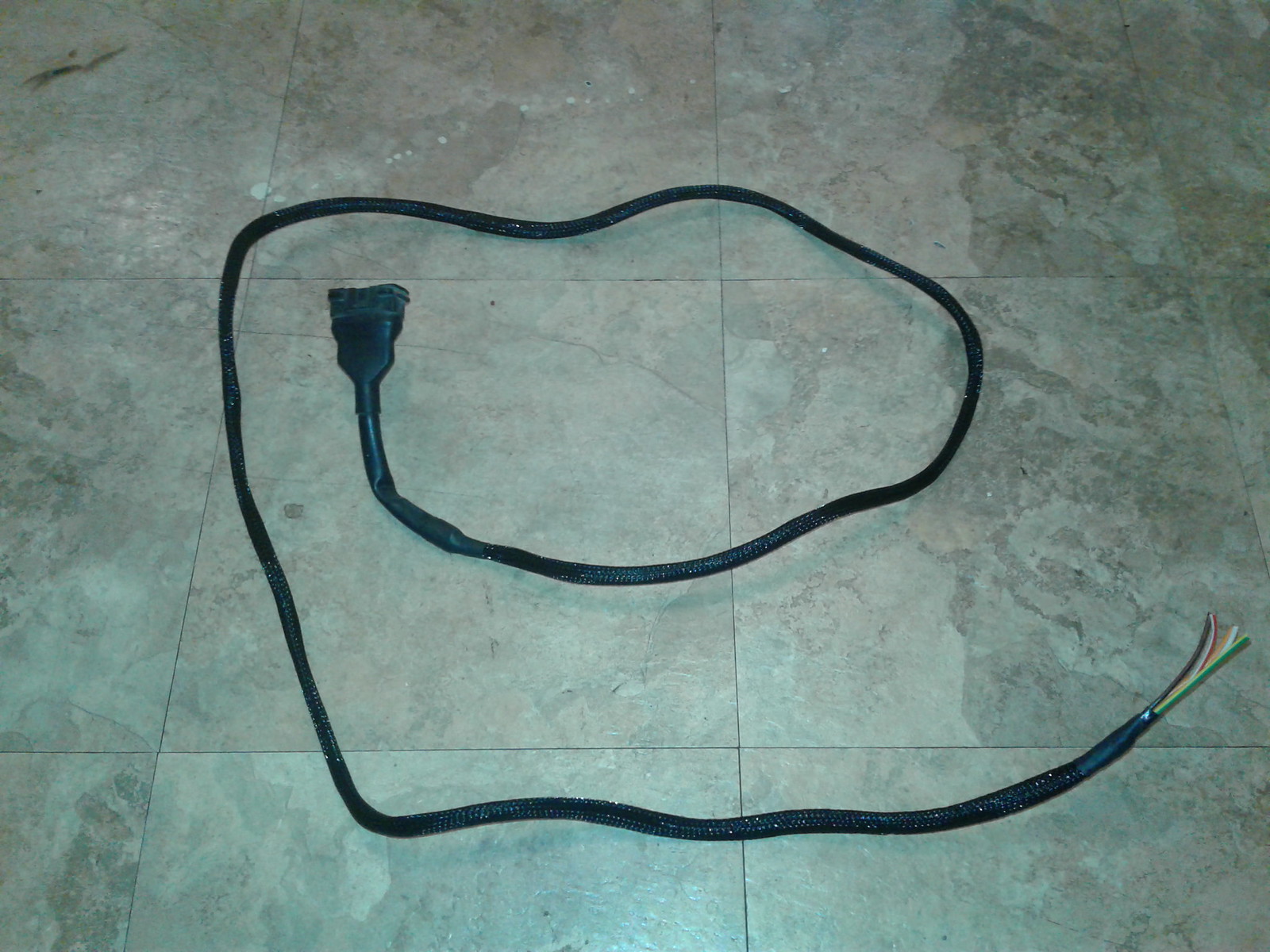This color photograph, taken in landscape orientation, captures a white marble tile floor composed of approximately six to nine 12-inch tiles, viewed from above. At the center of the image lies a broken black electrical cord, intricately coiled upon the floor. The coiled cord begins with a receptacle end devoid of prongs, accentuated by some black electrical tape. This end is slightly left of center. The cord spirals outward in a loop, moving to the right, then toward the top, back around to the left, and across the bottom. In the bottom right corner, the cord's sheath has been peeled back to expose a bundle of frayed wires in vibrant colors like yellow, green, red, and black, splayed in various directions. This image, with its detailed textures and colors, presents a realistic and representational view of a mundane yet intriguing scene.